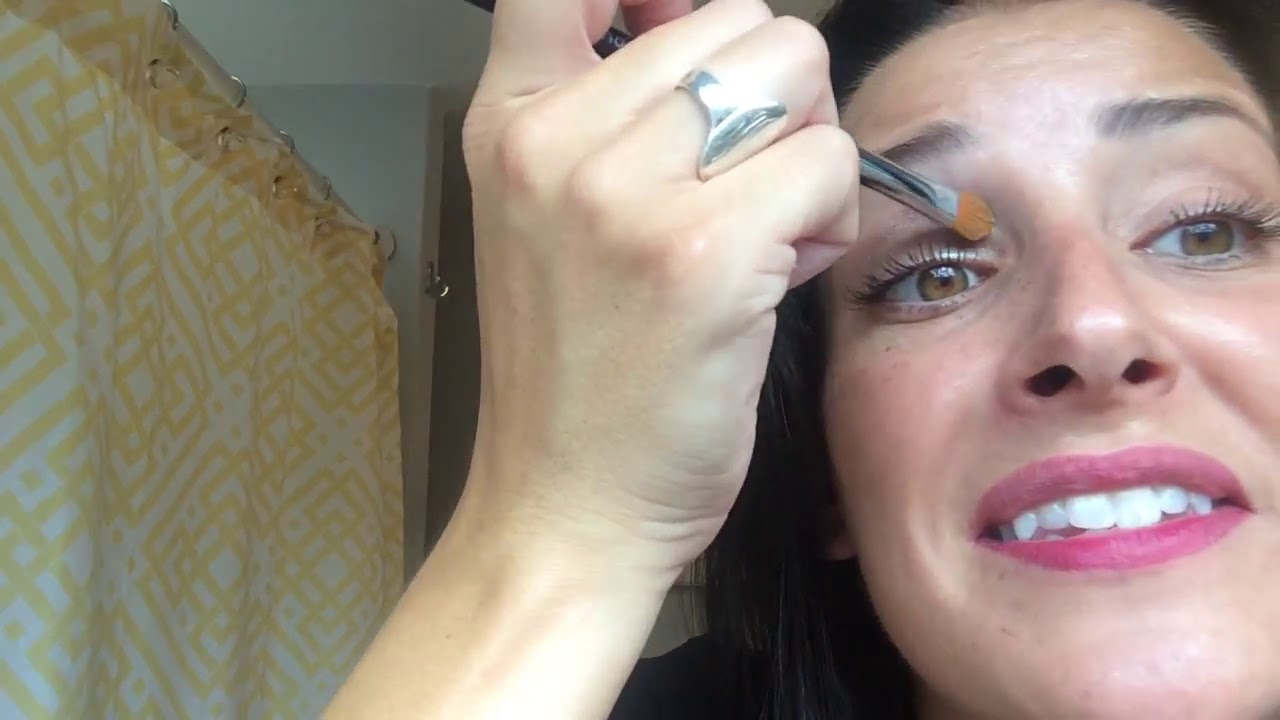In the image, a Caucasian woman with long black hair and brown eyes is applying makeup, possibly eyeliner, using her right hand. She has thin black eyebrows and bright pink lipstick on her slightly open mouth, revealing perfectly white but somewhat uneven teeth. She is holding a makeup brush with a light brown brush head and a silver handle. The woman's ring finger, which bears a silver ring, steadies the brush as she applies the makeup to her upper eyelid. Her mouth is open, and she appears to be in the midst of a tutorial or demonstration within a bathroom setting. To her left, there is a white wall and a shower curtain featuring a pattern of white and yellow squares and diamond shapes. To the right of the shower curtain, a small doorway is visible. The overall scene captures an intimate moment of detailed, personal beauty care.